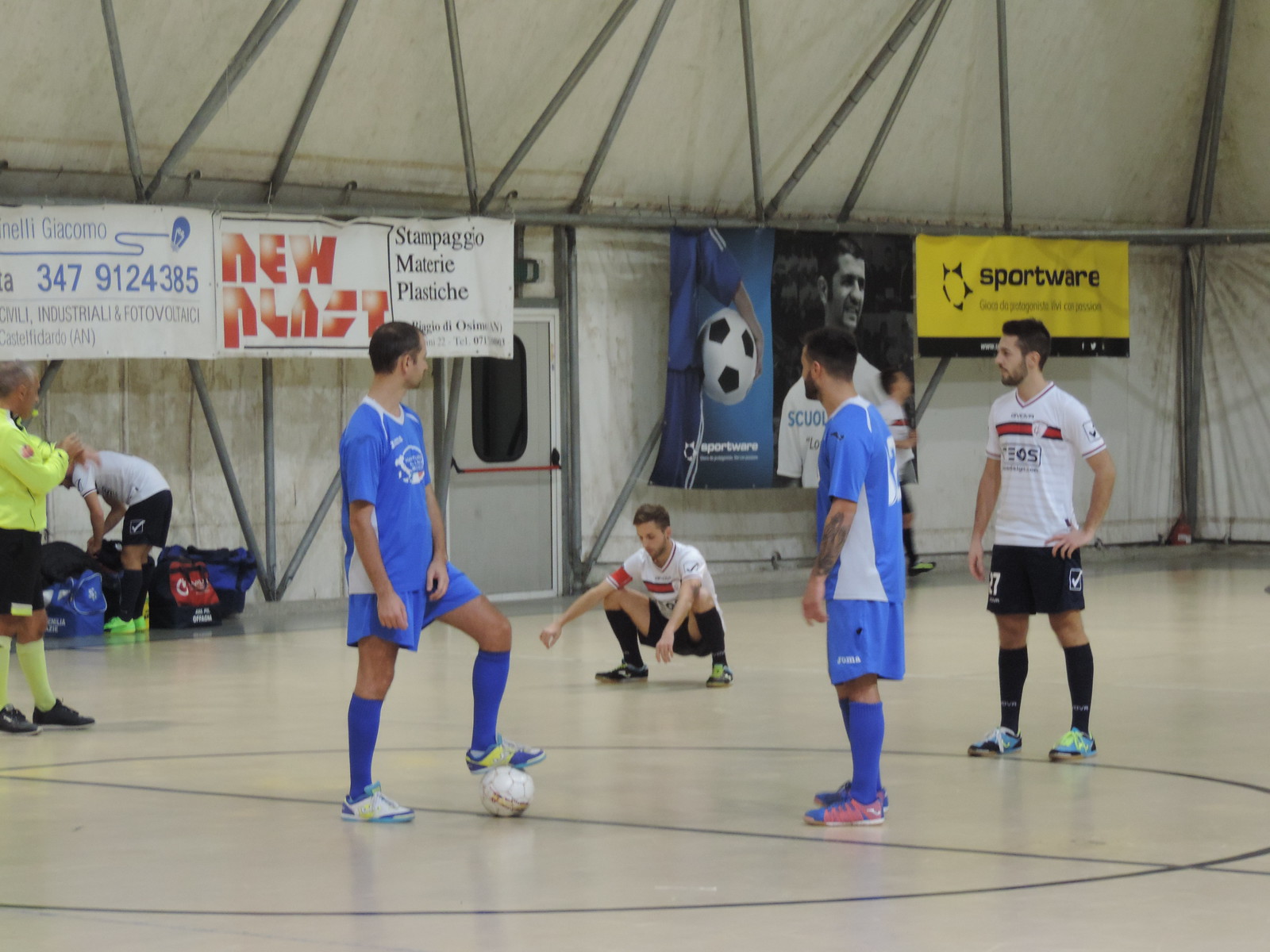In this rectangular image of an official indoor soccer game, both teams are positioned at the center of the court, which is a hard tan surface marked with long lines. The team in blue uniforms consists of players wearing blue shirts, shorts, and socks, adorned with blue, white, and yellow shoes. Notably, one of these players is standing with his foot on a white soccer ball, looking over his shoulder at another player in a crouched stance. The opposing team members are dressed in white shirts with black shorts and socks. To the left, a referee dressed in green and black oversees the action. The surrounding indoor setting features metallic framework, a doorway, and various signs in the background, including advertisements for local Italian businesses, indicating that the venue is in Italy. The backdrop consists of white drapery supported by metal beams, adding to the indoor ambiance.